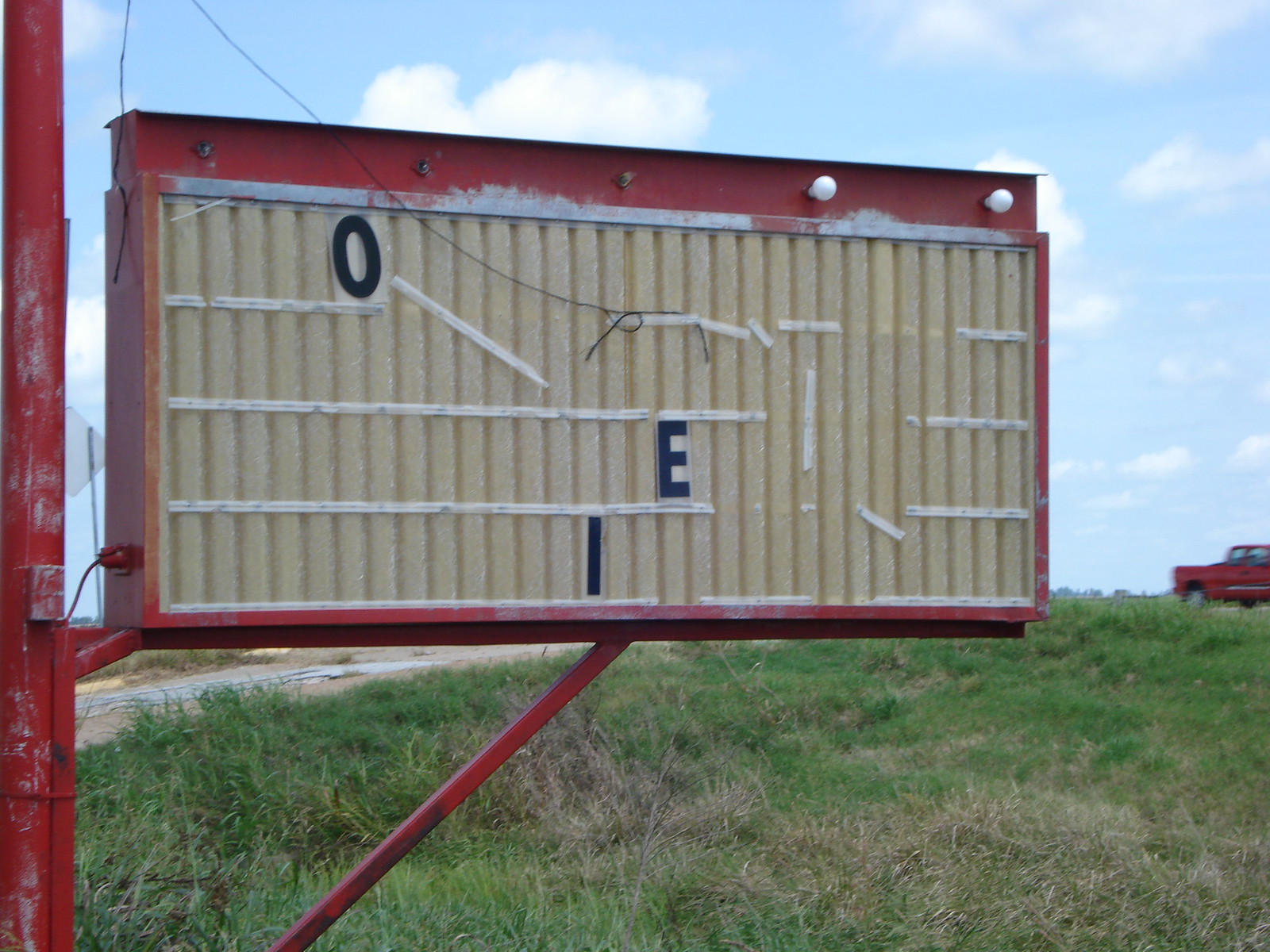A captivating photograph capturing a dilapidated sign standing resolutely in the middle of an expansive countryside. The vintage sign, painted red and mounted on a red post, features faded cream lettering reminiscent of old marquee signs that once announced upcoming acts in town. The sign is severely weathered, with only a few intact letters remaining—an "O" at the top, an "E" below, and an "I" further down. Its once vibrant paint is now chipped and discolored, speaking volumes of its age and neglect. The backdrop features an overgrown field lush with greenery and scattered weeds, suggesting many seasons of abandonment. To the side, a red pickup truck is parked on what appears to be private property, potentially a farm that the sign once advertised. The sky overhead is a pristine blue, dotted with fluffy white clouds, adding a serene contrast to the scene. In the distance, a gravel driveway winds away from the sign, hinting at former activity. Notably, the sign's framework still holds two out of five original light bulbs, long since extinguished, which once illuminated its message, adding a sense of nostalgia and faded glory to the image.